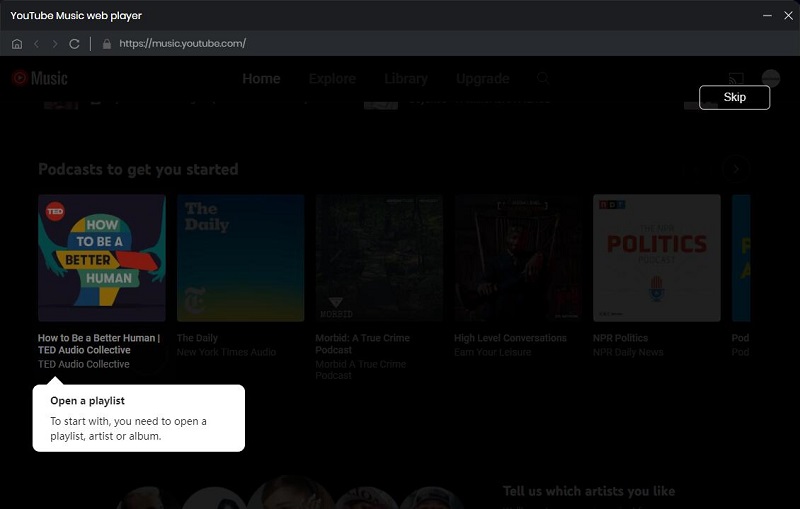This image captures a screenshot from a YouTube Music web player. In the top-left corner, the YouTube Music logo is prominently displayed in white font. The overall visibility is slightly obscured due to an on-screen pop-up message that appears within a speech bubble. 

In the lower section of the screen, there's a highlighted video titled "Podcasts to get you started," featuring a prominent TED logo in a white, uppercase font set within a red circle. The accompanying thumbnail depicts a pair of hands arranging puzzle pieces to form a human head. Beneath this thumbnail, the text "How to Be a Better Human" is displayed in white, followed by the attribution "TED Audio Collective" which is repeated.

The pop-up speech bubble at the bottom of the screen contains instructional text that reads, "To start with, you need to open a playlist, artist, or album." In the background, other content squares are faintly visible, adding depth to the interface.